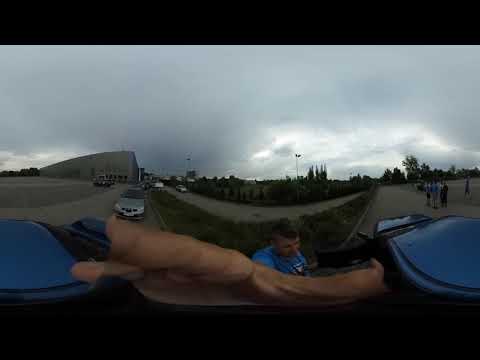The photograph captures an outdoor setting, likely from the vantage point of someone driving down a roadway or racetrack. Dominating the center of the image is a man with dark hair, dressed in a blue shirt, who appears to be looking downward. This man is in the foreground, with parts of his arms or hands visible, which might be due to the panoramic style of the photo. On the left side of the image, a silver or bluish car faces towards the camera, while other vehicles are scattered around the scene. In the background, you can see a curved track or roadway with some cars and pedestrians visible on the right side. There's a gray building or possibly a factory with loading docks on the far left. The sky is overcast and gray, casting a gloomy light over the area. Trees and vegetation line the horizon, adding depth to the landscape. Overall, the image is cluttered with elements that give it a slightly chaotic feel, with some details blurred or pixelated.